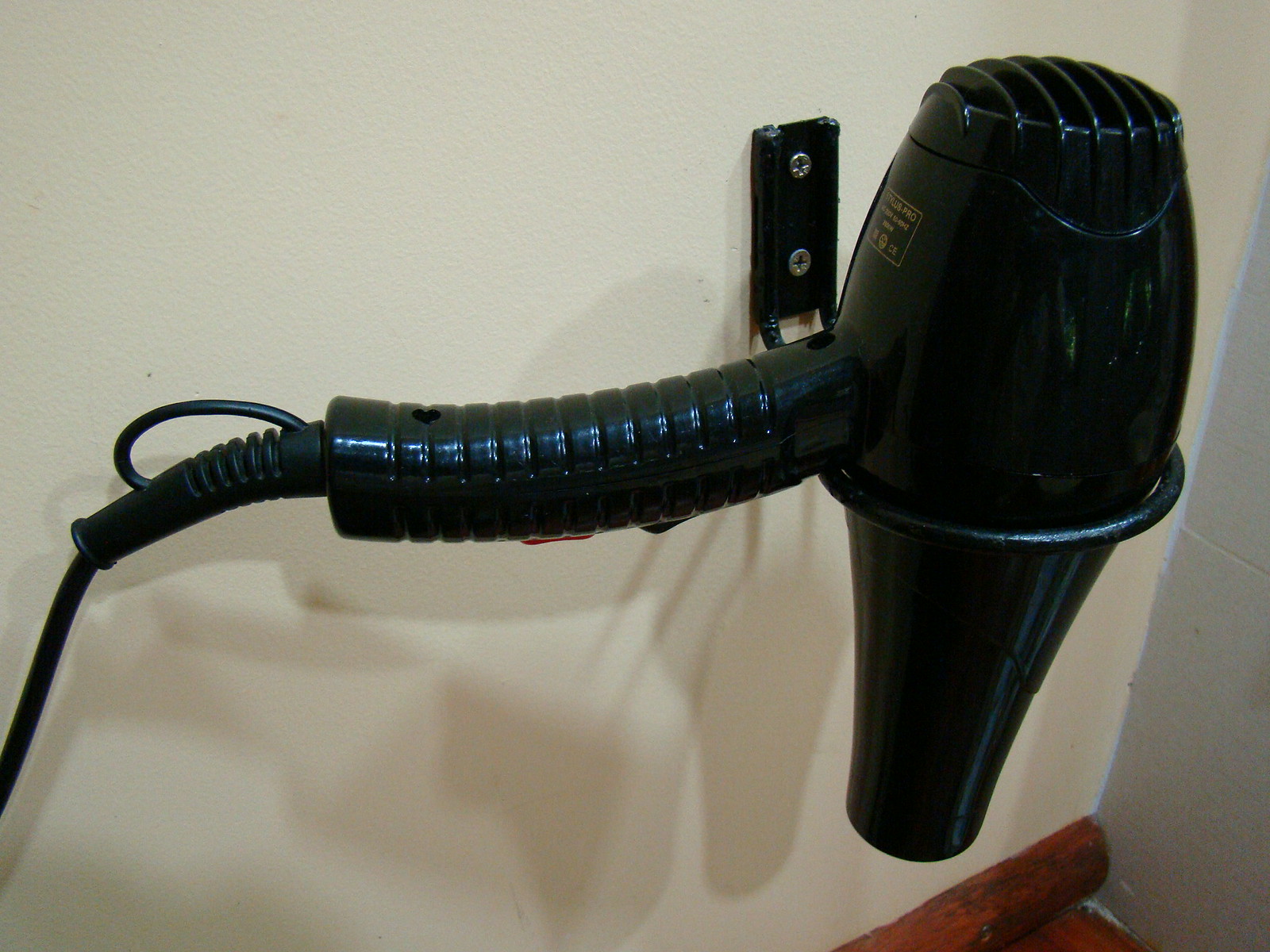The tightly cropped colour photograph features a black plastic hairdryer mounted on a metal ring attached to a light yellow, almost magnolia, smooth wall. The hairdryer, which has a black flex cable extending toward the bottom left of the image, is supported by a black backplate secured to the wall with two visible silver star screws. The handle of the hairdryer is long and rigid, with a red switch visible on it, and some indistinct gold lettering near the rear. The wall hosting the backplate casts a shadow, adding depth to the image. To the right side of the frame, a tiled wall with off-white tiles edging out of view, hints at a possible bathroom setting. At the bottom right corner, a reddish-brown wooden trim detail, potentially the edge of cabinetry, runs horizontally off the image, reinforcing a warm, commercial, or home-like setting.